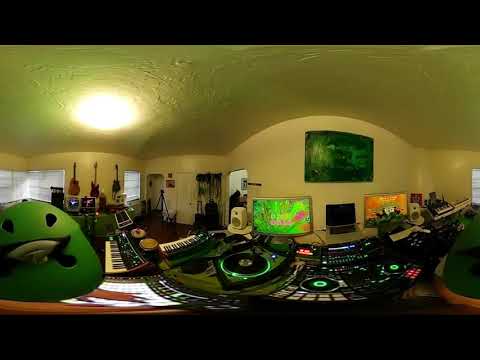The image depicts the panoramic interior of a musician's home studio, characterized by white walls and ceiling, creating a bright and well-lit atmosphere. On the left wall, three guitars are prominently displayed above a couple of keyboards. The room also features a central hub of activity with a large electronics board, adorned with numerous lights and buttons, flanked by monitors and a laptop between them. Scattered throughout the space are additional musical instruments, including multiple keyboards and a turntable, indicative of DJing equipment. A green and black painting adds a splash of color to the pristine environment. The shot appears slightly distorted due to the panorama mode, and a partial glimpse of a person is noticeable in the bottom right corner, adding a subtle human presence to the otherwise equipment-filled room.